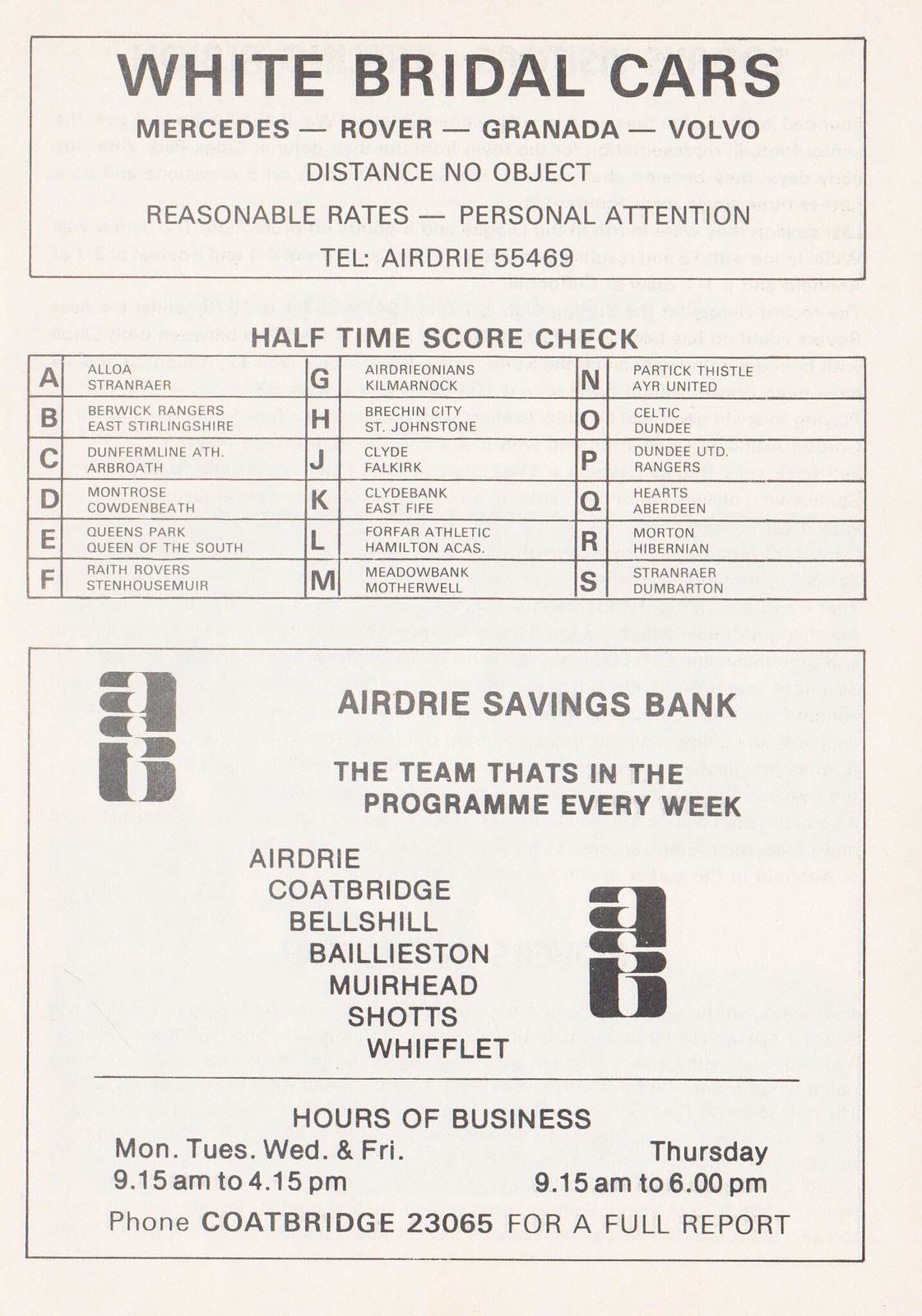The image is an old advertisement, likely from the 1960s or 1970s, featuring black bold text on white paper. At the top, it prominently displays information for a rental car service offering white bridal cars, including Mercedes, Rover, Granada, and Volvo. The advert emphasizes that distance is no object, provides reasonable rates, and guarantees personal attention. A phone number is listed for contact: G55469.

Below this, the advertisement features a section for "Halftime Score Check," with letters ranging from A to S, each corresponding to various names or locations (e.g., A: Aloha, Stranraer, B: Berwick Rangers, East Stirlingshire). This section seems to offer a service related to sports score updates.

Further down, the ad includes promotions for the Airdrie Savings Bank, described as "the team that's in the program every week," with locations like Airdrie, Coatbridge, Bellshill, Baillieston, Muirhead, Schatz, and Wifflet. Bank business hours are also listed: Monday, Tuesday, Wednesday, and Friday from 9:15 a.m. to 4:15 p.m., and Thursday from 9:15 a.m. to 6 p.m. 

Overall, the design and typography give a vintage feel and suggest the dual purpose of advertising both a car rental service and a local bank, combined with sports-related updates.